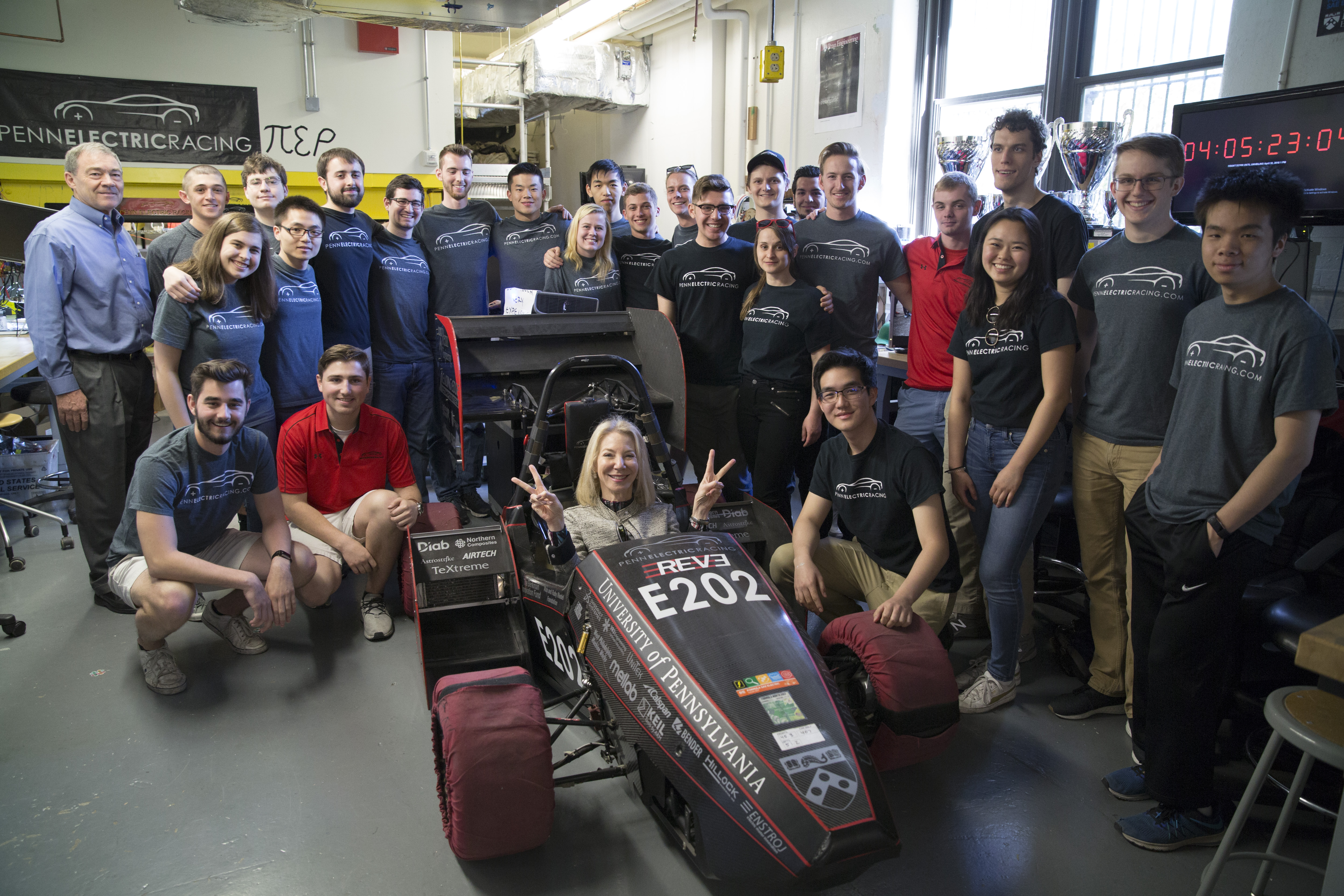A large group of around 26 or 27 people, comprised mostly of men with several women, is gathered in a spacious workshop, all facing the camera for a group photo. The individuals are either standing or kneeling, all smiling and posing for the camera. Most of them are wearing medium-gray t-shirts emblazoned with a white car logo and the words "Penn Electric Racing." In the center of the image, a woman with blonde hair is seated in a racing buggy with red wheels, marked "E202, University of Pennsylvania." She is holding up both hands in a peace sign. Behind her, the group is standing and kneeling, and a large banner on the wall displays the same "Penn Electric Racing" logo that is on their t-shirts.